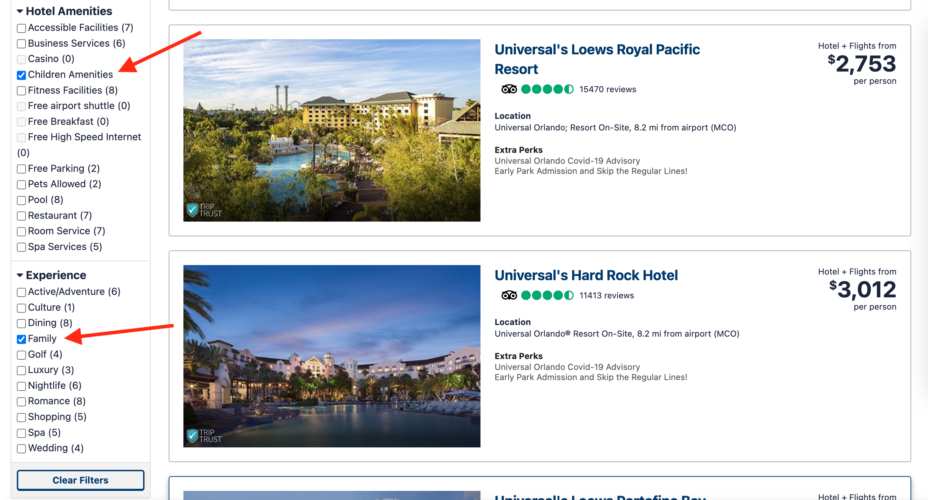This screenshot compares two hotels located in Universal Orlando, displaying key details and prices for each. The first hotel, Universal's Loews Royal Pacific Resort, has a guest rating of 4.5 stars from 15,470 reviews. It offers multiple perks, including early park admission and the ability to skip regular lines. The hotel is currently promoting a COVID-19 advisory. Packages including hotel and flights start at $2,753 per person.

The second hotel, Universal Hard Rock Hotel, also boasts a 4.5-star rating. Situated onsite, it is 8.2 miles from the airport. It provides similar extra perks: early park admission, skipping regular lines, and a COVID-19 advisory. The package price for hotel and flights is listed at $3,012 per person.

On the left side of the screen, amenities are detailed, particularly highlighting those for children and families with blue check marks, influencing the pricing based on selected preferences and needs.